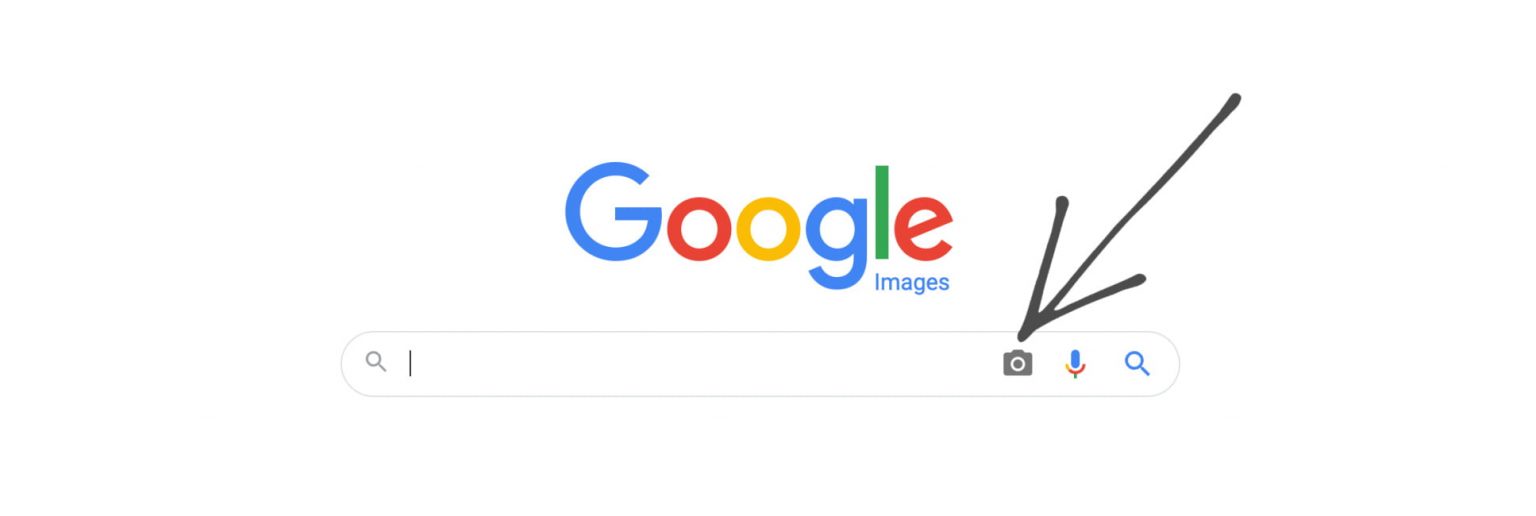The image features a clean white background with the Google logo prominently centered. The iconic logo is composed of a blue capital "G," followed by lowercase letters: a red "o," a yellow "o," a blue "g," a green "l," and a red "e." Positioned beneath the "l" and "e" of "Google," the word "Images" appears in blue, starting with a capital "I" and followed by lowercase letters.

Below the logo is a long rectangular search bar designed for image searches. On the left side of the search bar, there is a small magnifying glass icon representing the search function. An active cursor line is present within the bar, indicating where users can type their queries. 

To the right side of the search bar, there are three distinct icons: a grayish-black camera symbol, representing the image upload search function, followed by a blue and red microphone icon for voice search. The microphone is blue at the top, features a red semicircle, and has a small blue line beneath it. Adjacent to the microphone is another blue magnifying glass icon, echoing the search function.

A black arrow is pointing downward from the top of the image towards the camera icon, emphasizing its presence.